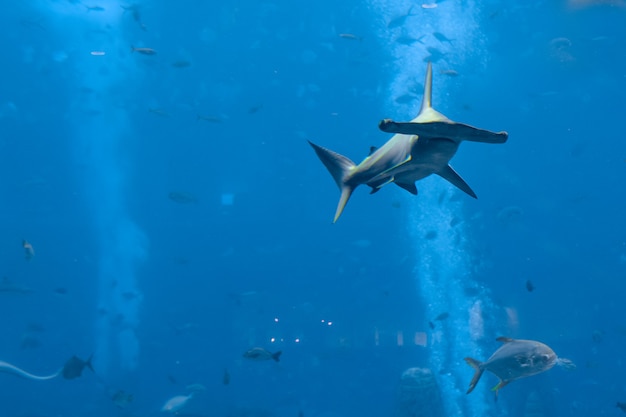This captivating underwater image, likely taken deep in the ocean or possibly in an aquarium, showcases the mesmerizing marine life in a very dark blue expanse of water. Light filters through the water in streaks of lighter blue on both the left and right sides, providing a serene backdrop to the scene. Small fish of various sizes and species swim throughout the background, adding to the aquatic ambiance.

Dominating the foreground is a striking hammerhead shark, positioned near the upper center of the image. Its long, distinct hammer-shaped snout is immediately eye-catching, accompanied by a sleek, dark gray body, pointed top fin, and two smaller fin arms below. This graceful predator appears to be swimming towards the photographer but slightly off to the side, creating a dynamic focal point.

In the bottom right corner of the image, another prominent fish, possibly another species of shark, is visible. This large, grey fish has an oval, more robust structure, distinguishing it from the hammerhead. Together, these marine creatures create a compelling and detailed snapshot of underwater life.